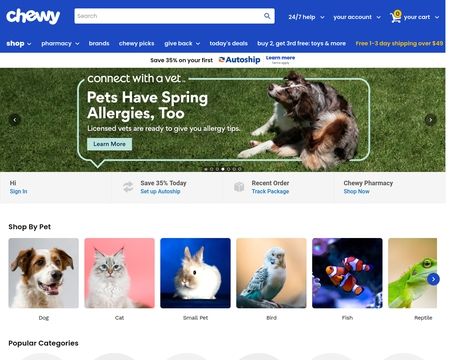Homepage Overview for Chewy Website:

The homepage of Chewy’s website features a visually appealing and user-friendly layout predominated by a blue theme. At the very top, a vivid blue horizontal bar spans the screen, imparting a vibrant and welcoming atmosphere. Positioned in the top-left corner, the playful Chewy logo is prominently displayed in white text, juxtaposed with the website’s name in a fun, inviting font.

To the right of the logo, a sleek white search bar is embedded, inviting users to "search" via the gray placeholder text within. The search bar is punctuated on its right edge with a classic magnifying glass icon. Adjacent to the search bar, the user finds a 24/7 Help drop-down menu, easily identifiable by an accompanying white downward arrow. Following this, there is another menu option for account settings, also marked with a corresponding white arrow.

Next in line is the cart symbol, highlighted by a circular yellow badge containing the number "0" in black text, indicating an empty shopping cart. To the immediate right, one finds an additional cart drop-down menu for swift access to cart details.

Below this primary navigation, a series of secondary menus allows users to explore various sections of the site. From left to right, these include:
- **Shop** (with a drop-down arrow, currently in bold),
- **Pharmacy**,
- **Brands**,
- **Chewy Picks**,
- **Givebacks** (with a drop-down arrow),
- **Today's Deals**,
- **Buy 2, Get 3rd Free**,
- **Toys & More**.

On the far right, eye-catching yellow text proclaims "Free 1-3 day shipping over $49."

A thick white dividing line follows, prominently displaying the offer "Save 35% on your first AutoShip" in the center. Next to this, an icon resembling a refresh button (or share button), with an orange downward arrow and a blue upward arrow, is accompanied by the blue text "AutoShip." Below, additional text prompts the user to "Learn more," though two smaller gray words beneath are indistinct.

The main image below this section unfolds against a grass background, reading "Connect with a vet" in bold text within a partial rectangular box. Inside this box, the larger text states "Pets have spring allergies too," while smaller script explains, "Licensed vets are ready to give you allergy tips." An action button within prompts visitors to "Learn more." Complementing the text is a picture of a dog lying in the grass.

Directly beneath this are interactive buttons including:
- Hi (grey button),
- Sign In (blue button),
- Share Button,
- Save 35% Today (grey button),
- Set Up AutoShip (blue button),
- Recent Orders panel with an icon of a box and blue text "Track Package",
- Chewy Pharmacy section with blue "Shop Now" text.

At the bottom lies a singular row of "Shop by Pet" options, each represented in a square with a thematic stock photo for different pets:
- Dog (brown ears and white fur against a gray background),
- Cat (white cat with a pink background),
- Small Pets (either a gerbil or bunny with a blue background),
- Bird (white parakeet with a beige background),
- Fish (two clownfish with a dark blue background and a piece of coral),
- Reptile (green lizard with a tan background).

The row concludes with a blue circular arrow icon allowing users to scroll right.

Across the very bottom, partially visible, are more options for popular categories, indicated by the tops of gray semicircles resembling a series of domes.

This detailed description conveys a thorough layout of the Chewy website homepage, illustrating the visual components and interactive elements designed to enhance user engagement and navigation.